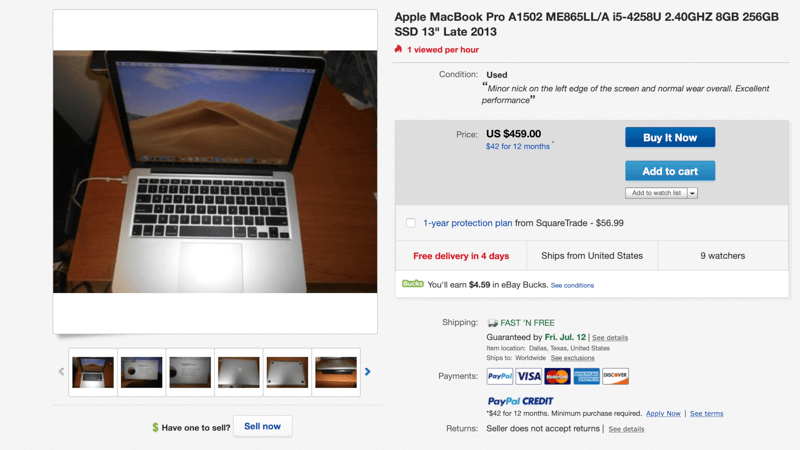This image portrays an online listing, likely from a platform such as eBay, showcasing an Apple MacBook Pro. At the upper right corner, there is a large, clear image of the MacBook displaying the Mojave Desert background on its screen, accompanied by a Mac keyboard. The laptop is viewed from above, plugged in, and resting on a wooden desk.

To the left of the main image is the detailed description of the product. The listing specifies an Apple MacBook Pro model A1505, with a 13-inch screen from the year 2013. The product information is presented in black text. Below this, in red text, it indicates that the item is viewed approximately once per hour. The condition of the laptop is marked as used, with a note that there is a minor nick on the edge of the screen but it offers excellent performance.

The price is listed at $459, with a financing option of $42 per month for 12 months. Two call-to-action buttons are visible: a dark blue "Buy It Now" button with white text, and a slightly lighter blue "Add to Cart" button, also with white lettering. Additionally, there is a dropdown menu related to a one-year protection plan from SquareTrade, suggesting that SquareTrade might be the protection service provider rather than the selling platform.

The listing mentions free delivery within four days, shipping directly from the United States. It is guaranteed to arrive by July 12th. Various payment options are available, including PayPal, Visa, MasterCard, American Express, Discover, and PayPal Credit.

Below the main image are several more images, including screenshots of the MacBook in use and a close-up of the minor nick on the side, providing potential buyers with a comprehensive view of the product's condition and functionality.